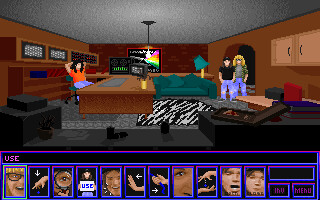This image appears to be a screenshot from a computer game reminiscent of the early '90s era, possibly inspired by classic films or shows like "Wayne's World" or "Bill and Ted." The setting is a detailed, cartoonish room that evokes the look of a motel living room, characterized by brown or dark red walls and a leopard-print carpet. At the center of the room stands a long rectangular wooden table. To the right of the table is a small blue couch, near which a man and a woman are seen standing in front of an arch-like doorway.

Further details include a figure sitting at a large desk on the left side of the image; this character, possibly a woman in an orange shirt, has her arms folded behind her head. The character design suggests a casual setting, enhanced by a relaxed pose. The scene features additional elements like terminals, hinting at a recording studio or office environment rather than a typical living room.

At the bottom of the image are several smaller, bordered squares, outlined in purple and blue, displaying various body parts of different individuals, possibly indicating character selection or interaction points. This complex and vibrant depiction captures the quirky and laid-back atmosphere of the game, blending elements of homey comfort with a professional vibe.